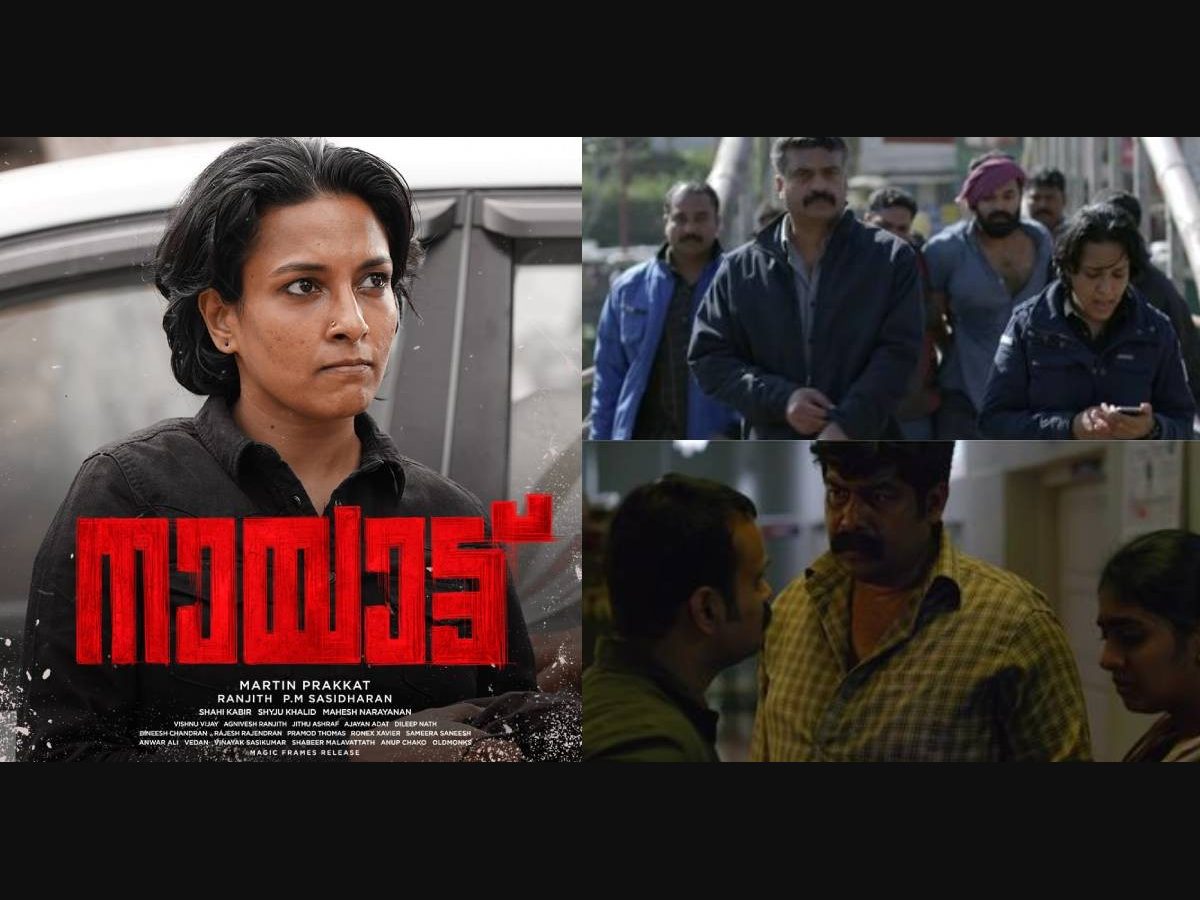This collage is composed of three distinct images, set against a black background, suggesting it might be a movie poster. On the left, there is a photograph of a woman who appears to be Indian, characterized by her short dark hair, parted down the middle, and adorned with a nose ring and earrings. She is looking up to her left with a slightly irritated expression. She is wearing a black button-down shirt, and behind her, a vehicle is visible. Accompanying this image is some red and white text, presumably in an Indian language, including names like Martin Prakat and Ranjith PM Sastryan.

To the right, there are two stacked images. The top image portrays several people, likely also Indian, crossing a bridge while clad in dark blue clothing. One of the females in this group is looking down at a phone-like device. The bottom image is darker and depicts a large man in a yellow checkered shirt conversing with another man, while a girl looks on with a displeased expression. The darker tones and indoor setting of this photograph contrast with the relatively brighter outdoor scene above it. Overall, the collage conveys a narrative with its blend of distinct yet interconnected scenes, embodying the essence of a movie poster.